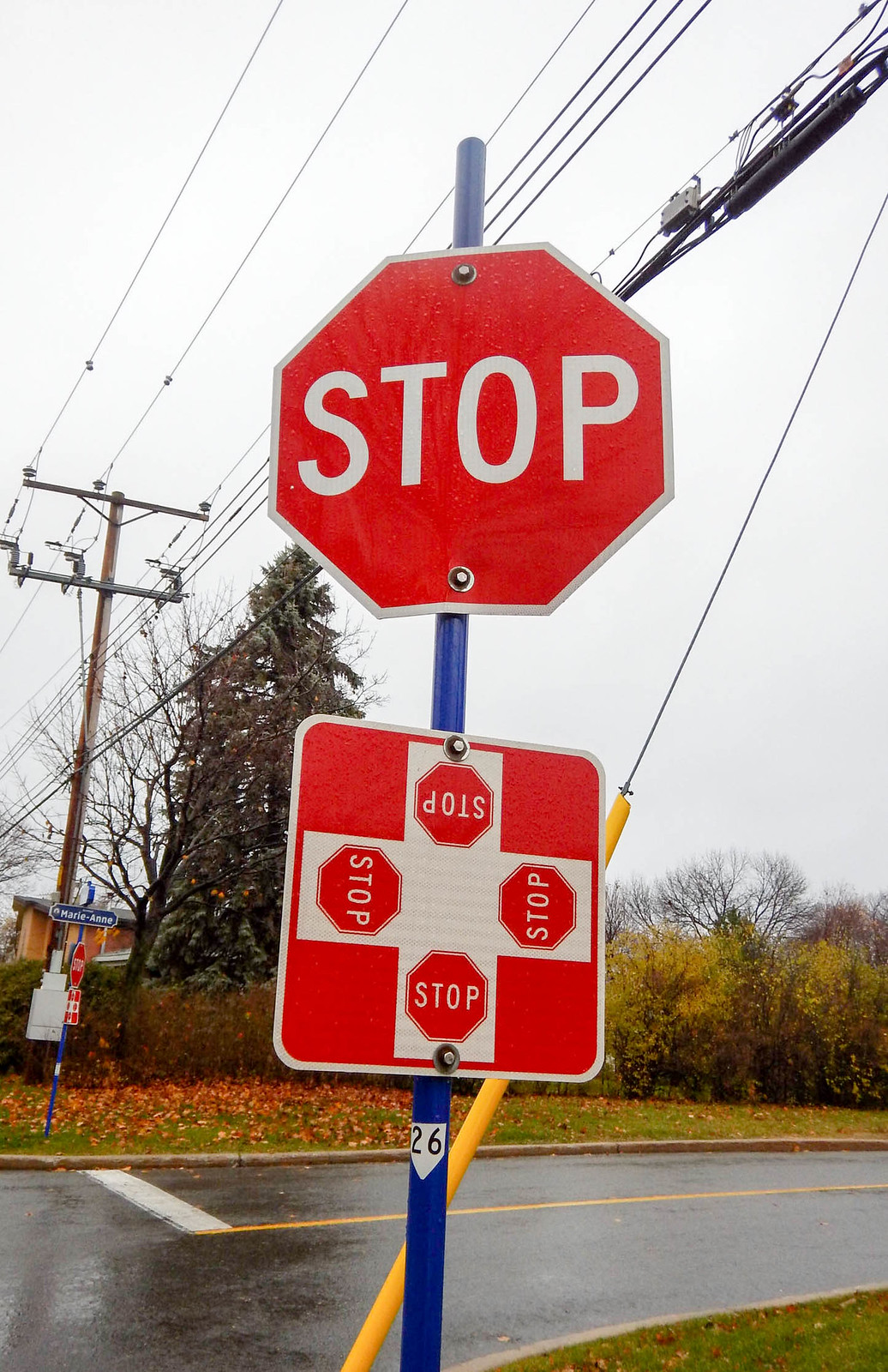This photograph captures a slightly upward view of a busy intersection dominated by a prominent stop sign on a blue pole. At the top of the pole is a standard red and white stop sign, and directly beneath it is a smaller square sign featuring four miniature stop signs arranged in a white cross, indicating a four-way stop. The pole is also marked with the number 26. Overhead, electricity cables stretch across the gray sky. In the background, trees and grass frame the scene, and a small house can be seen in the distance. A secondary stop sign, accompanied by another smaller sign, marks the far side of the intersection. The roads are tarred, with visible yellow and white lines, and the grass appears neatly cut. The street name "Marie d'Anne" is indicated on a sign in the background.